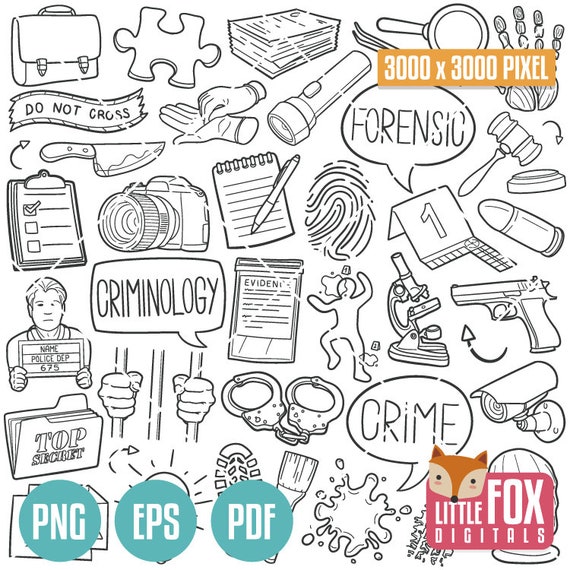The image in question is a meticulously organized square collage composed of numerous smaller icons, predominantly rendered in black and white. Among these icons are various clip-art illustrations including a puzzle piece, camera, clipboard, "criminology" sign, notepad, fingerprint, calendar, bullet, gavel, flashlight, pair of gloves, and a magnifying glass, among others, collectively hinting at a theme related to criminology or detective work.

In the upper right corner of the image, there's an orange box containing white text that reads "3000 by 3000 pixels," signifying the image's resolution. Moving to the bottom left, three circular icons in blue feature white text labels: the leftmost circle says "PNG," the one to its right says "EPS," and the one almost at the center says "PDF," likely indicating the available file formats of the image.

In the bottom right portion, a reddish box marked with the white text "Little Fox Digitals" is prominent, with a fox head emblem adorning the top edge of this box, symbolizing the brand associated with the design.

This detailed caption provides a comprehensive visual and functional overview of the image, suitable for clear representation.